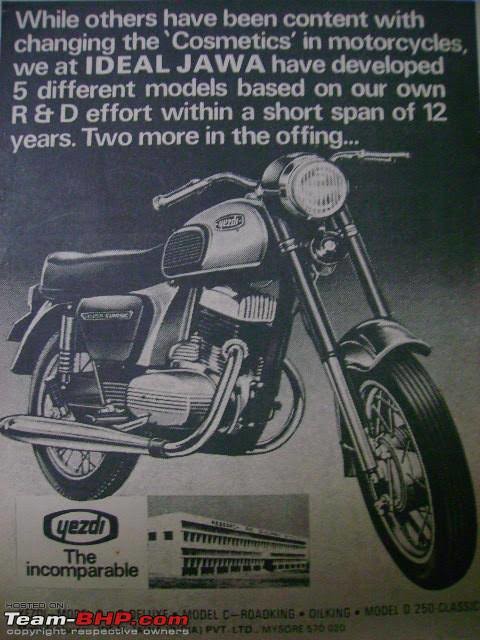This black-and-white magazine advertisement features a hand-drawn illustration of a vintage-style motorcycle positioned in the center with its front wheel slightly tilted to the right. Above the motorcycle, white text reads: "While others have been content with changing the cosmetics in motorcycles, we at Ideal Jawa have developed five different models based on our own R&D effort within a short span of 12 years. Two more in the offing..." Below the motorcycle, bold text spells out "YEZDI the incomparable," accompanied by a drawing of a building. In the bottom left corner, a watermark in white and red font states "team-bhp.com," alongside the note "copyright respective owners."